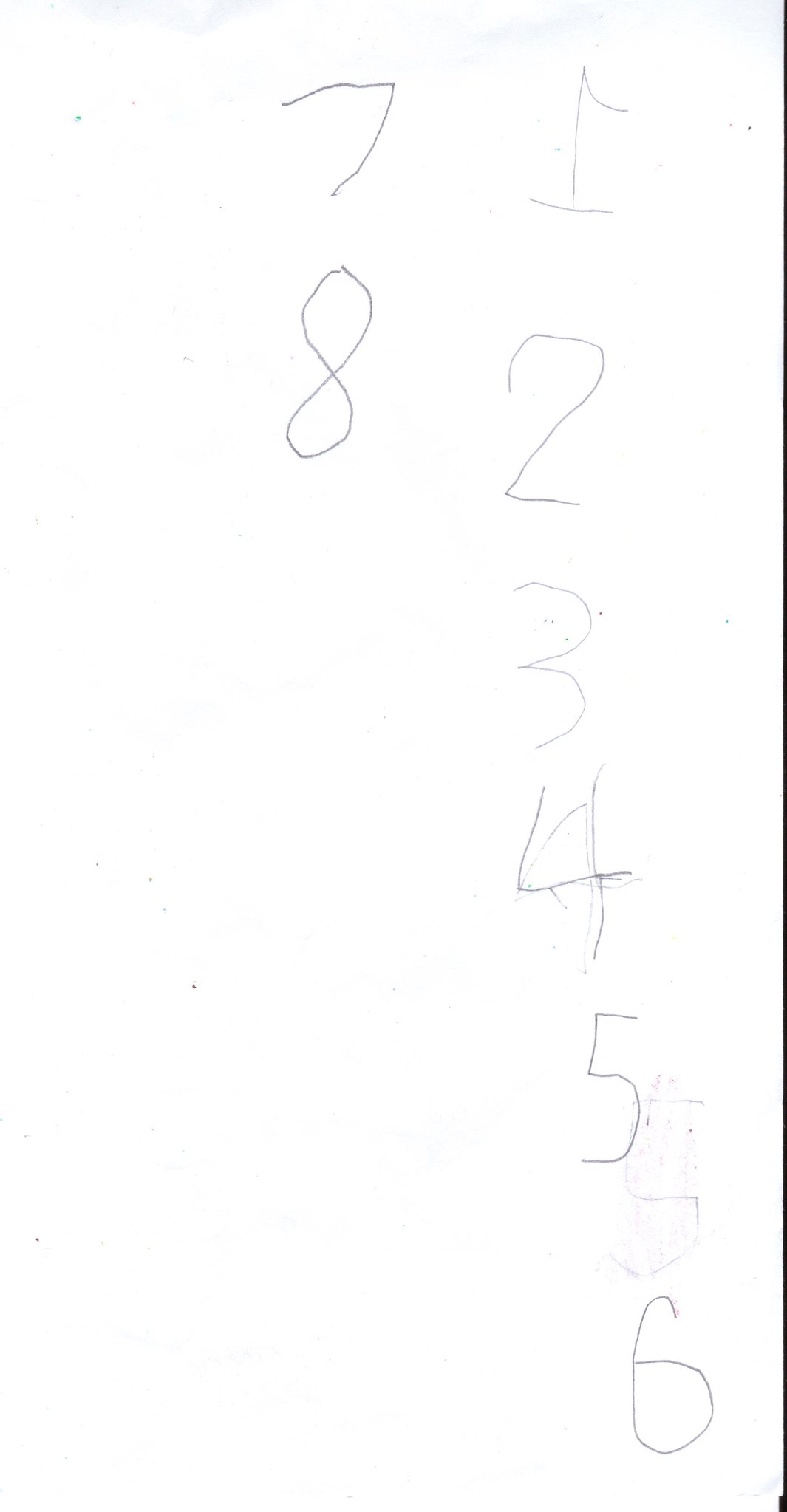The image displays a white surface, either a piece of paper or a wall, covered with pencil-written numbers. Centrally and towards the top, there is a noticeably crooked number seven, directly beneath which is an eight. To the right of these numbers is a vertical column of digits. The top of this column features a backwards number one, with the small part of the one facing right instead of left. Directly below the one is a two, followed by a three, and then a four. The four has a small smudge connecting the horizontal and vertical lines. Continuing down, there is a five, with an erased yet still visible five to its lower right. Finally, a six is situated at the bottom of this column.